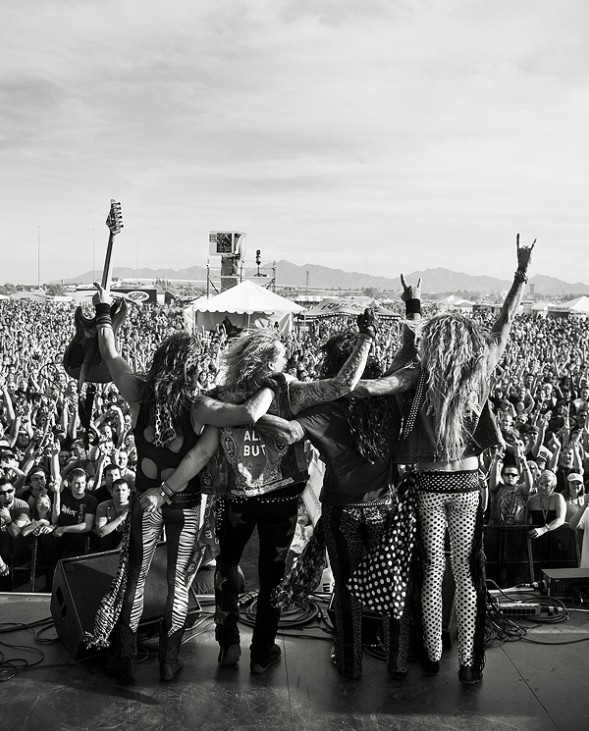In this black and white photograph, a heavy metal band commands the stage at an open-air concert, captivating a massive crowd against a backdrop of distant mountains and a cloudy gray sky. The scene is electric with enthusiasm as the sea of fans raises hands and waves energetically. The band consists of four members, each distinguished by their unique style and presence. 

On the far left, a tall, slender figure strikes a pose, holding up an electric guitar with their left hand. They sport polka-dot pants and a matching bandana hanging from their left pocket. Next to them, a band member with zebra-striped pants and a black, hole-ridden vest lifts their right hand in the iconic rock sign. This individual, with highlighted brown hair, stands confidently, contributing to the overall fierce look of the group.

The second member from the left is a striking figure with long, curly blonde hair. They wear a denim vest emblazoned with the partially visible text "L...B U T" and flaunt a tattoo sleeve on their right arm, which is raised in the rock sign. Completing their edgy look, they have leather gloves and dark shoes.

On the far right, another member donning see-through, fishnet stockings and a black vest waves their right hand in a peace sign. Their blonde hair cascades down their back, reaching mid-waist.

The band, with their hands raised in unison flashing the iconic rock hand signs, overlook a vast crowd and a white tent in the center, flanked by speakers and structures possibly housing sound equipment. The atmosphere captured in the photograph exudes the raw energy and unified thrill of the live heavy metal experience.